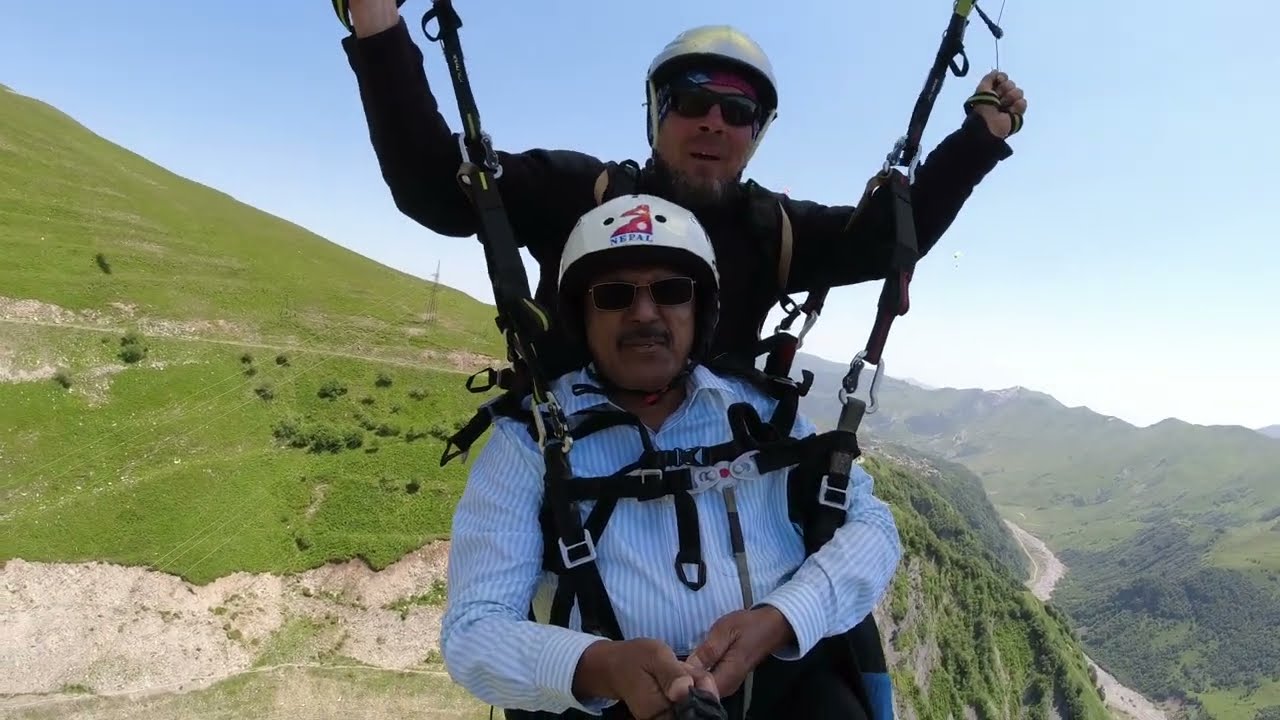The image captures two men in mid-air, likely during a skydiving or paragliding adventure. The man in front, wearing a blue and white striped shirt and a white helmet adorned with a red design and the Nepal flag, is holding a selfie stick and has a mustache. The man behind him, controlling the parachute with his arms raised, is dressed in a black long-sleeved jacket and a white helmet, sporting both a beard and a mustache. Both men wear sunglasses and are securely harnessed together with visible buckles and straps. In the background, a lush green valley features prominently, with a flowing river to the right and a mountainous, tree-covered area to the left under a clear blue sky.